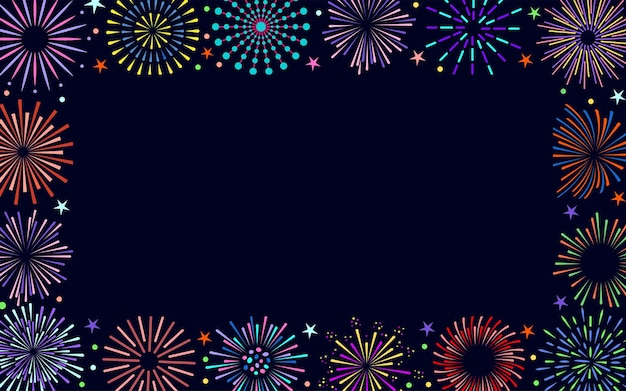This is a colorful and vibrant digital image designed as a border or background, ideal for wallpapers or a PowerPoint presentation. The backdrop is an extremely dark blue, almost black, and it is adorned with various symmetrical fireworks exploding along all four sides, creating a festive frame. There are a total of 16 fireworks, with six on the top, six on the bottom, and four distributed on the sides, including the shared corner ones. Each firework is unique though they have similarities in color palettes. 

From left to right in the top row, the fireworks include combinations such as pink and purple, yellow and blue, light blue with red dots, pink and purple again, blue and light blue with purple, and a mix of yellow, purple, and pink. The left side features a red and pink firework, while the right has an orange and blue one. In the left part of the third row, there’s a pink and purple firework, and on the right side, a green and orange one. The bottom row from left to right showcases fireworks in green and purple, red and pink, an intricate pattern combining light blue, blue, pink, and purple with green, red, purple, and blue circles, another yellow and purple, a lighter shaded red and pink, and finally green and blue.

Adding to the lively display, between the fireworks, are small multicolored stars and dots. The overall style is cartoonish with flat, bold colors. The fireworks feature a variety of patterns, including lines and circles, evoking a sense of celebration reminiscent of a firework show or a festive holiday like the 4th of July. This detailed, festive border creates a vibrant and happy visual effect, filling the edges of the deep blue space.